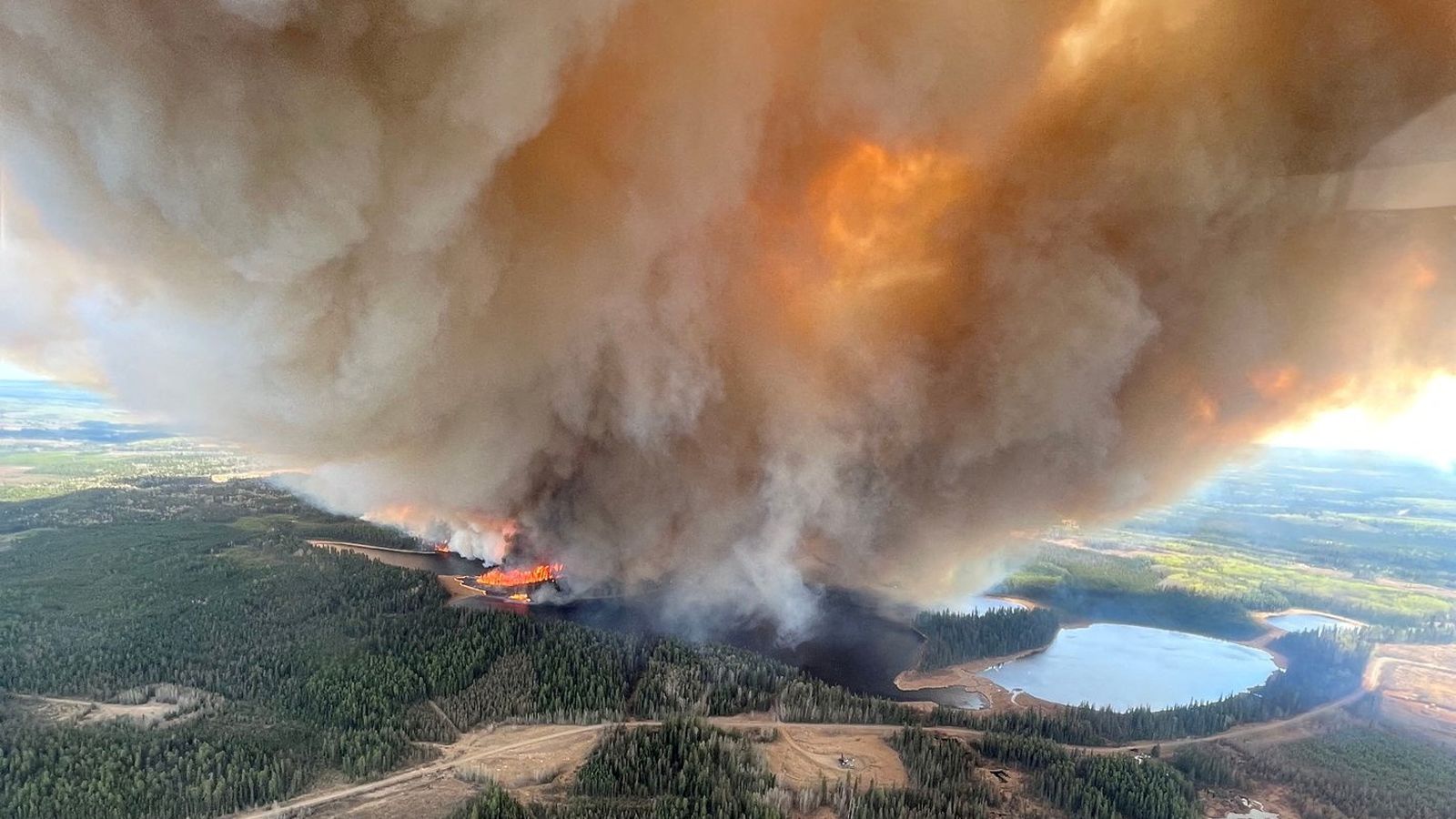This photograph captures an astonishing aerial view of a massive forest fire in a daytime setting. The central focus is a gigantic, billowy plume of grayish-brown smoke that stretches across the entire image from the left to the right edges. The thick smoke obscures much of the sky, save for a fiery orange glow piercing through its center, hinting at the intense blaze beneath. Towards the bottom of the image, the forest area appears engulfed in vibrant orange flames. To the left of the forest, there is a round, light blue lake, bordered by a small dirt road that winds in front of it and around the woodland. Surrounded by countless trees, this depiction vividly showcases the destructive power of the fire amidst the natural landscape, under the undeniable brightness of a sunny afternoon.